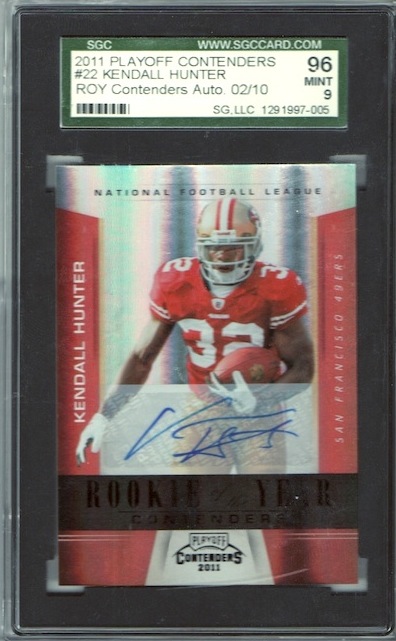The photograph showcases a meticulously encased football card of Kendall Hunter, evaluated by SGC, with their official website www.sgccard.com displayed at the top. This 2011 Playoff Contenders card has been graded mint 96 and is accompanied by a black background that frames the card. The card itself features a silver backdrop with red vertical stripes on each side, the left reading "Kendall Hunter" and the right "San Francisco 49ers." The header includes "National Football League," while the bottom red banner highlights "Playoff Contenders 2011." Kendall Hunter, wearing player number 32, is pictured in the center, overlaid with his autograph. Despite the card's mislabeling with number 22, it also includes a barcode, designation of "Roy Contenders Auto 02/10," and additional identification numbers beneath it.